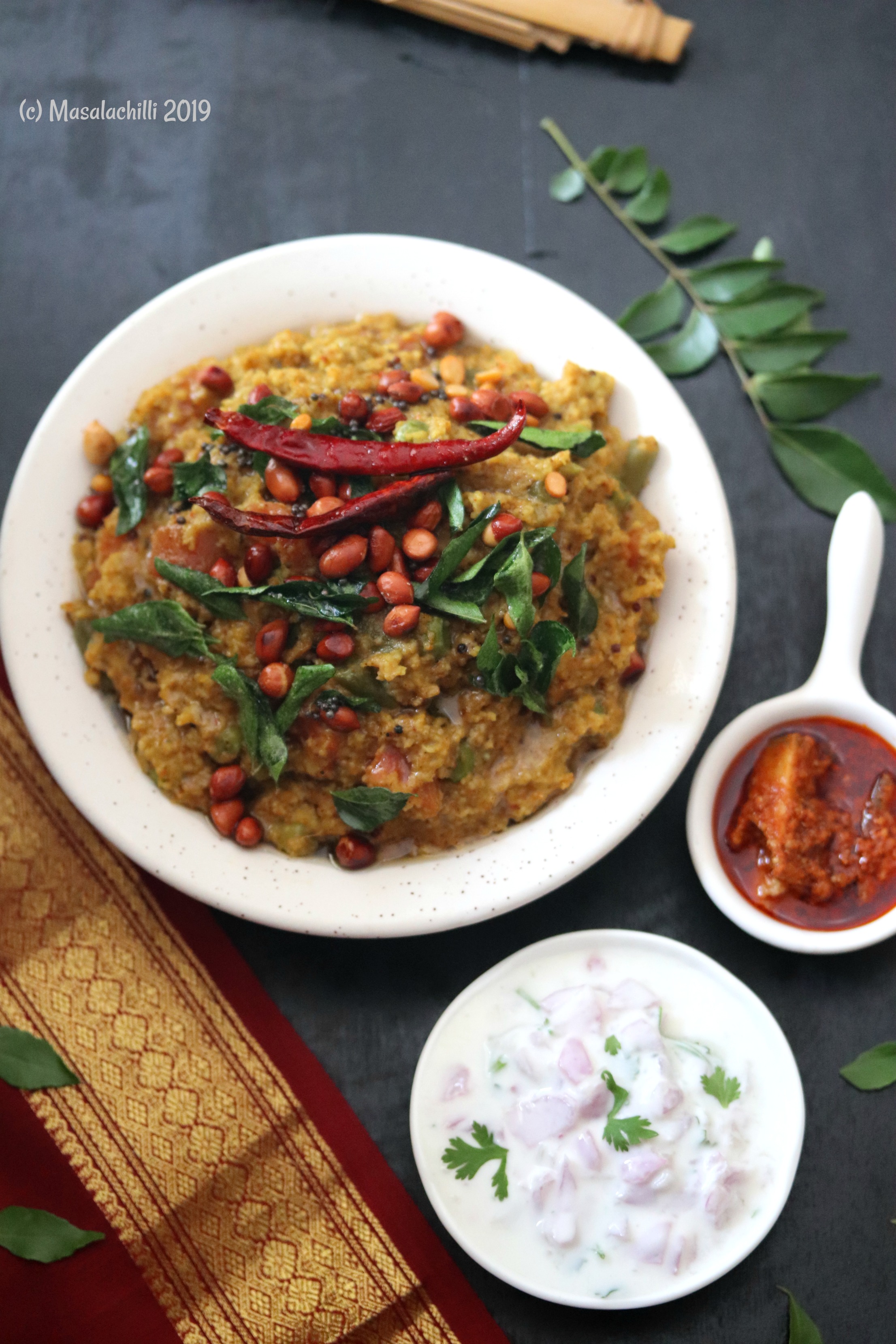The image captures a close-up aerial view of a rich, elaborate meal setting placed on a dark gray stone tabletop. Dominating the center is a large white plate holding a colorful, textured dish that appears to be a creamy, curry-style stew with a yellowish-brown hue. Within this main dish, there are roasted chickpeas and pinto beans scattered throughout, along with sprinkles of green leafy herbs, likely spinach, and two grilled red chili peppers adorning the top. To the right of the main dish, there are two smaller white bowls: one contains a thick red sauce with oily undertones and a chunk of food in the center, while the other holds a creamy white soup garnished with chopped onions and cilantro. The table is embellished with a luxurious deep red table runner featuring gold trims, and a stem of green foliage lies across the surface, adding a natural element to the ornate setting.